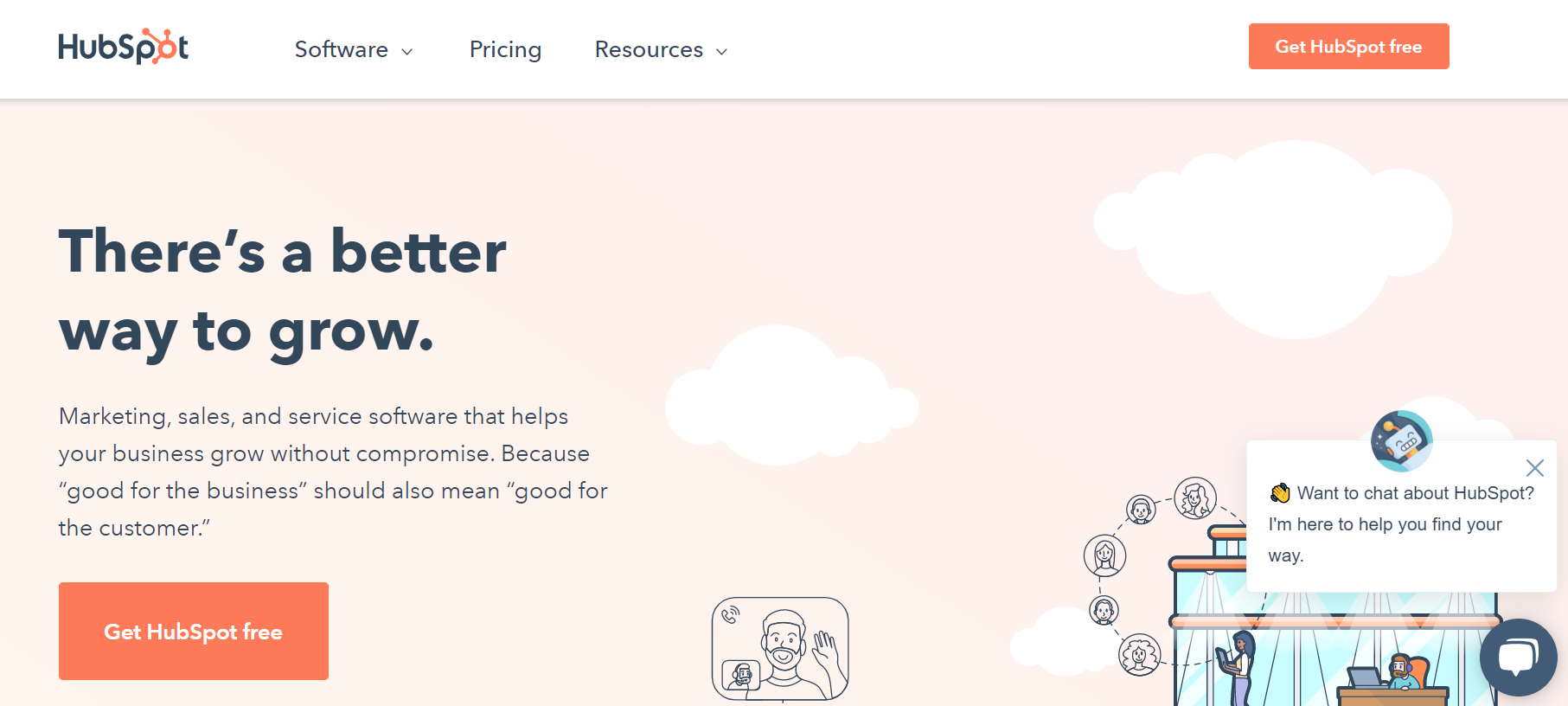A detailed and cleaned-up caption for the described screen capture:

"A monitor displays a screen capture of HubSpot's website. At the top left, the HubSpot logo is prominently featured on a white background in black and red font. Adjacent to the logo, three menu options—'Software' with a down arrow, 'Pricing,' and 'Resources' with a down arrow—are presented in black text. On the far right, an orange rectangular button with white text invites users to 'Get HubSpot Free.'

The website's desktop wallpaper is a very muted pink, adorned with lighter muted pink clouds drifting across the right-hand side. On the left side, in large bold black letters, the phrase 'There's a better way to grow' stands out. Beneath this headline is a succinct paragraph that reads, 'Marketing, sales, and service software that helps your business grow without compromise. Because "good for the business" should also mean "good for the customer."' In the bottom left corner, another orange button with white text offers, 'Get HubSpot Free.'

Center stage is a square icon featuring a line drawing of a man with fluffy hair and a beard, seemingly waving at the viewer. He appears to be wearing a headset, with a phone icon situated in the bottom left corner of the square. Adjacent to this, on the right-hand side, there's a circular image of a cartoon-style bot above the message, 'Want to chat about HubSpot? I'm here to help you find your way.' Below this, a blue image depicts someone seated at a desk working on a computer in cartoon style, with a woman standing to the left, holding a laptop."